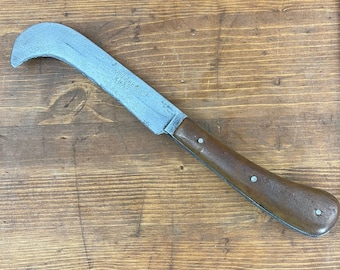This up-close photograph captures a handmade or amateur-made knife resting on a weathered, old wooden table. The table features a grainy texture with visible knots, markings, and dark brown scratches, giving it a rustic appearance. The knife's handle, positioned in the lower right of the image, is crafted from wood and shows signs of wear, with a smooth, rounded bottom. Secured with three silver metal rivets, the handle attaches to a steel gray blade that starts straight but curves into a hook-like shape towards the tip. The curved blade includes some unreadable engraving, adding a unique detail to the knife. The overall composition highlights the knife's craftsmanship against the backdrop of the aged wooden surface.